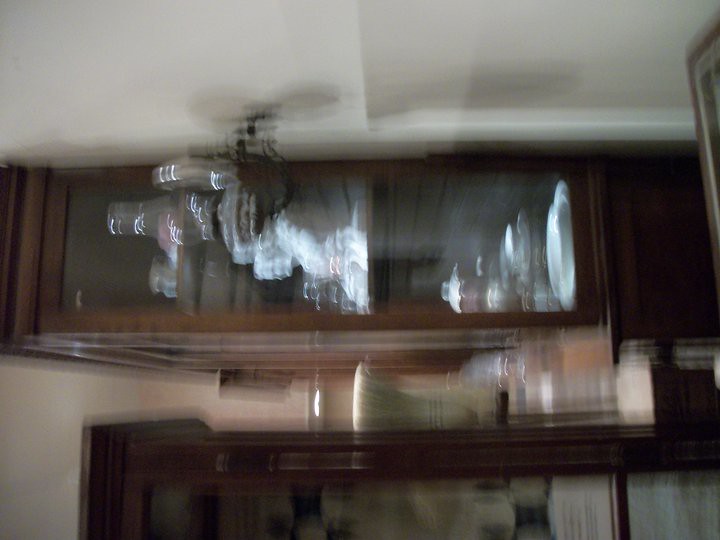This appears to be a very blurry image taken inside someone's house, with noticeable camera movement. Dominating the picture is a white, likely off-white ceiling, beneath which hangs a black light fixture with several bulbs. Centrally featured are two brown wooden cabinets with glass fronts. The top cabinet is long and rectangular, stretching almost across the entire width of the image, and is possibly attached to the ceiling. Below this top cabinet, separated by a visible space, is another similar glass-fronted cabinet. There is a broom positioned horizontally between these two cabinets, with its bristles visible in the middle of the picture.

Inside the top cabinet, reflections obscure clear visibility, but there appears to be glassware or similar items. The lower cabinet, described as a curio stand, contains several items, including what looks like dishes standing on edge, oil lamps, a statue, and some fine china. Additionally, there is a sneaker or something in a jar placed on top of the bottom cabinet. The overall blurriness of the image, along with the reflection from the light, makes it challenging to discern the finer details.